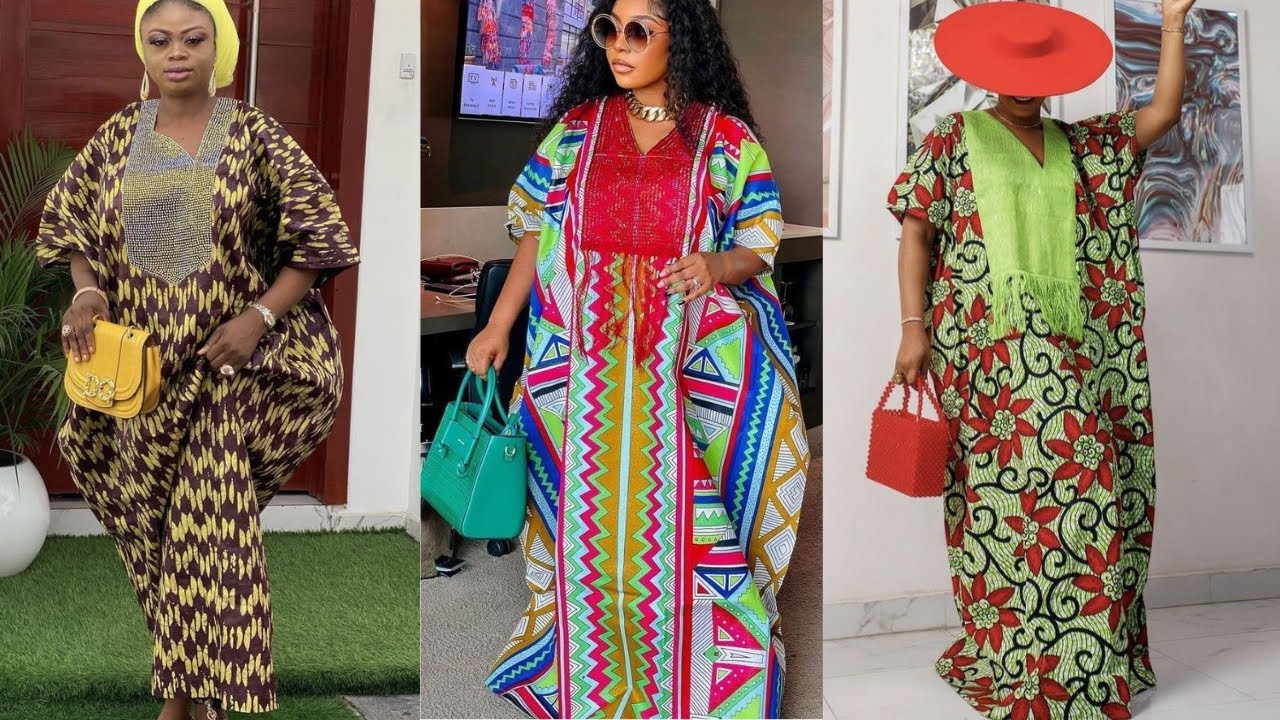In this image, likely a modeling catalog print or advertisement, there are three panels featuring African-American women showcasing vibrant African print outfits. 

The first panel on the left depicts a woman adorned in a yellow and black chevron-striped outfit, paired with a yellow headscarf, a gray t-shirt, and a yellow purse. She is posed against a backdrop of green grass and a doorway. Her outfit appears to be a loose, baggy ensemble, possibly with pant legs.

The middle panel features a woman with long, wavy hair who is looking to the side. She wears sunglasses, a gold necklace, and a red v-neck top layered with a colorful printed outfit imbued with shades of red, yellow, green, pink, and blue. She is holding a turquoise bag.

In the third panel on the right, another stylish woman is seen in a green dress accented with red floral patterns. She completes her look with a red wide-brim hat, a red purse, and a green scarf around her neck. The background hints at an indoor setting, possibly a home with artwork on the walls. This detailed and vibrant image emphasizes the diversity and richness of African print fashion.